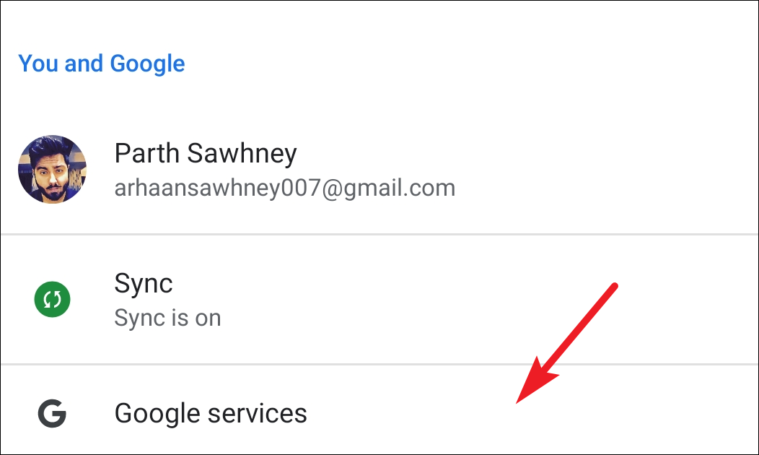The image depicts a user interface with several labeled sections. At the top, there is a square icon followed by the text "You and Google" in blue. Beneath this, the name "Path Swayne" appears, accompanied by an associated Gmail account: Arhansawhney007@gmail.com. Next to the email, there is a profile picture icon indicating it's a Gmail account. Below this, the interface displays the word "Sync," followed by "Google Services" at the bottom. An attention-grabbing red arrow points toward the "Google Services" section.